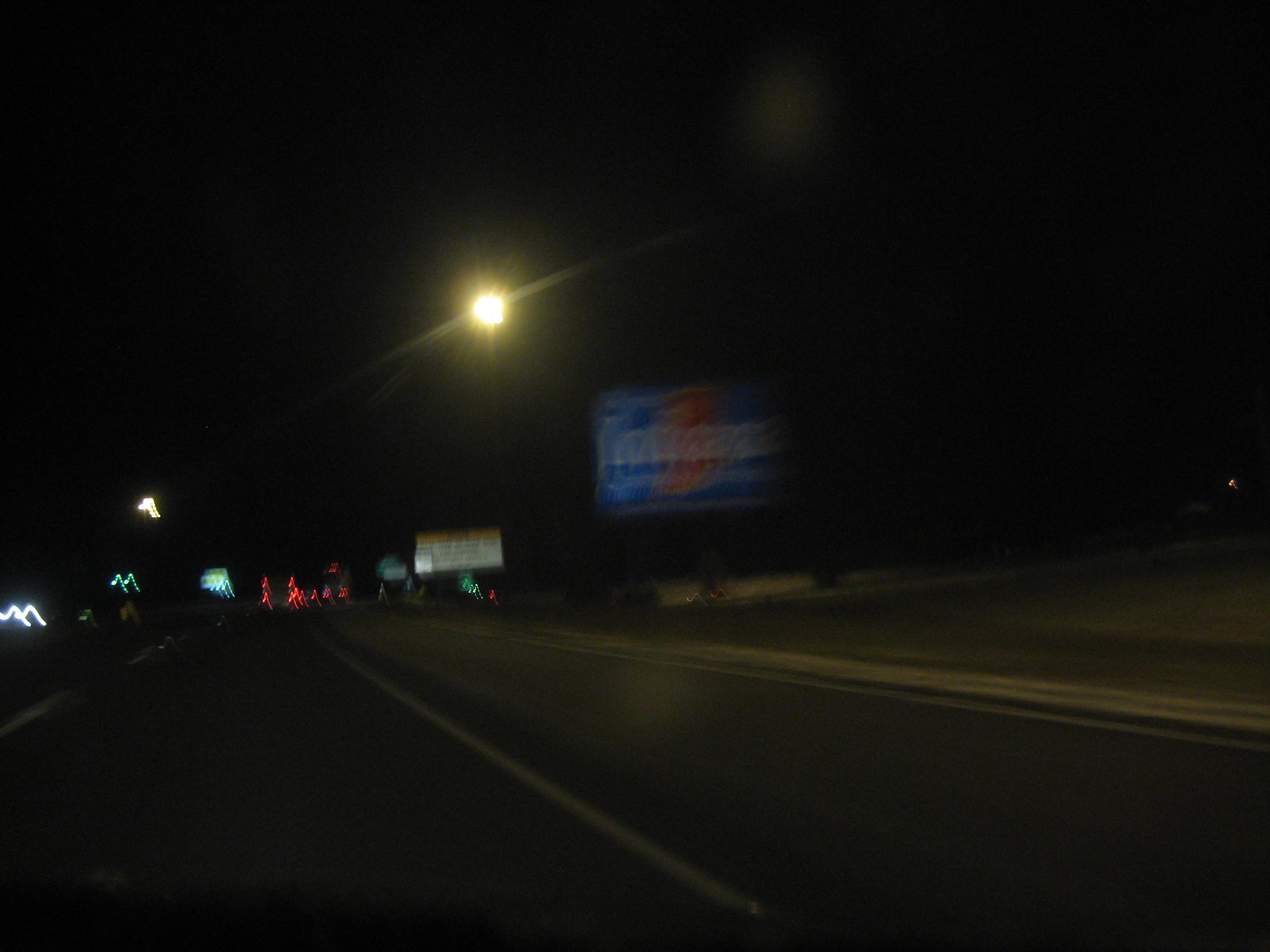This photograph, taken at night from inside a moving vehicle, is remarkably dark and blurry, giving the scene an eerie and indistinct appearance. The sky is pitch black, with a singular bright yellow dot, likely the moon, just left of center. The foreground shows a roadway with a faint white line, and a pair of red taillights from a distant vehicle. To the left, there are green and white triangular lights, likely from buildings. The right side of the road features a grassy area and a prominent blue billboard with an orange shape in the center, possibly saying "Tennessee." Additional signage includes a possible construction sign further back, topped by a bright streetlamp. Scattered across the image are streaks of dragged lights in green, blue, red, yellow, and white, enhancing the sense of movement and adding to the overall blurry quality.